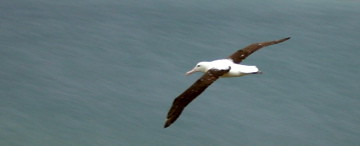This image captures a vibrant scene featuring a seagull in mid-flight over a body of water. The sky, predominantly blue with soft white streaks, has a delicate pinkish hue suggesting either dawn or dusk light. The seagull, prominently situated in the middle to right of the frame, glides effortlessly from right to left with its wings fully extended. The bird's body is white, accentuated by a tan beak and alert black eyes, while its narrow wings exhibit a contrasting brown shade. Below, the water mirrors the sky’s rich blue tones, enhancing the serene yet dynamic atmosphere of the photo. The seagull's positioning and spread wings convey swift movement, giving the viewer a sense of the bird's graceful flight across this tranquil, ambiguous body of water.